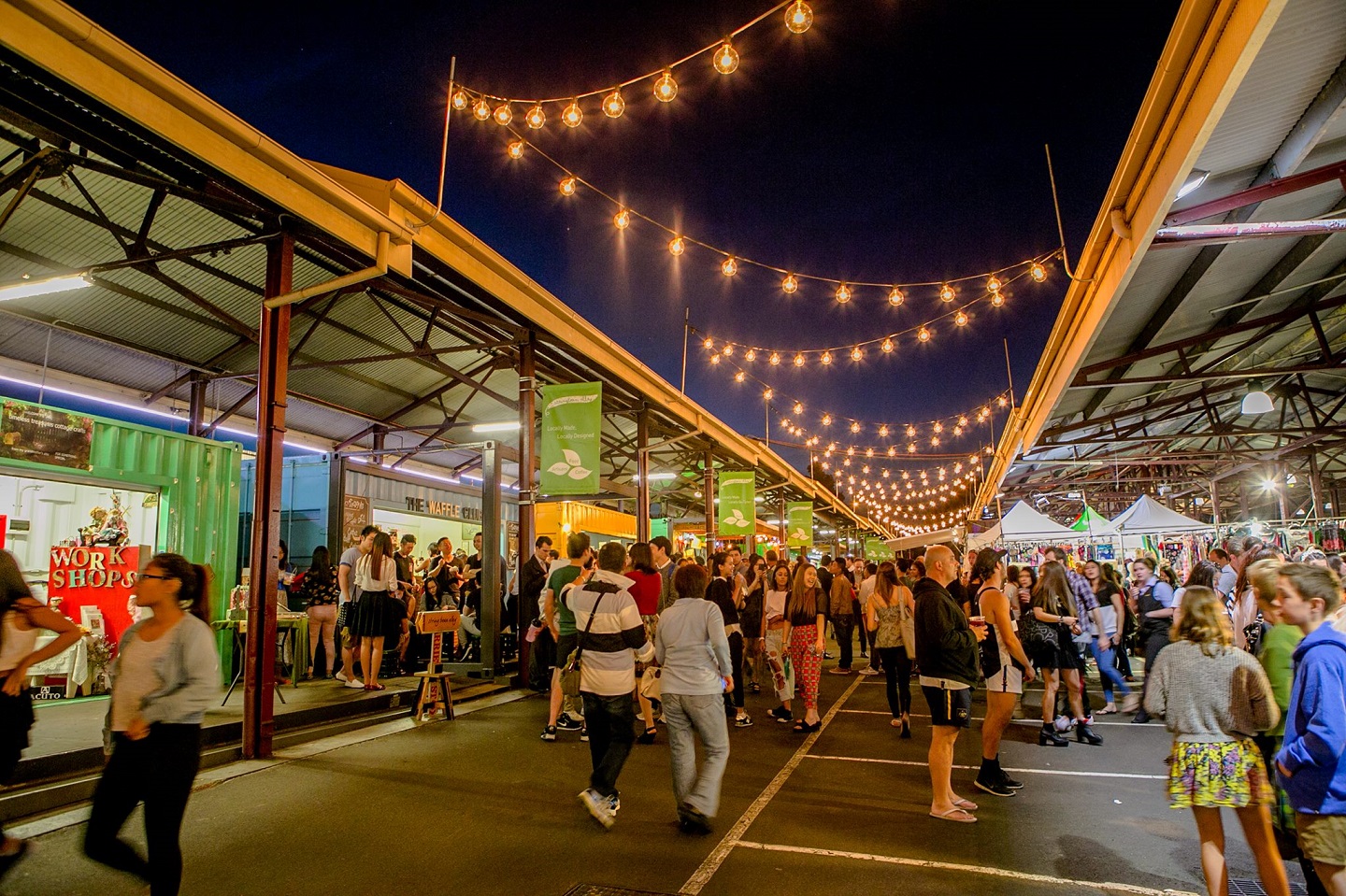This detailed photograph captures a bustling nighttime scene at the Queen Victoria Market in Melbourne, renowned for its lively night market. The image, presented in landscape orientation, showcases a vibrant outdoor market divided into two main areas on the left and right. Above each strip of shops, metal-framed awnings provide shelter for the numerous visitors milling about on the cement walkways below. The dark night sky is visible between these awnings, adorned with a multitude of lights strung in zigzag patterns, illuminating the market with a festive glow.

The shoppers are surrounded by a mix of retail setups, including white pop-up tents to the right and creatively repurposed shipping containers on the left, which serve as unique shops. These containers have been modified with cutouts to allow easy access for patrons. The market is lined with bright green signage on vertical posts, advertising locally made and designed products such as coffee and food. The street, devoid of vehicles, contains parking spaces along the right side. Additionally, a prominent yellow gutter or trim piece lines the awnings, creating a diagonal visual effect that leads the eye toward the market’s horizon.

Overall, the photograph is a splendid example of photographic representational realism, capturing the essence and energy of the outdoor market, where amateur business vendors and farmers converge to sell their diverse array of wares.